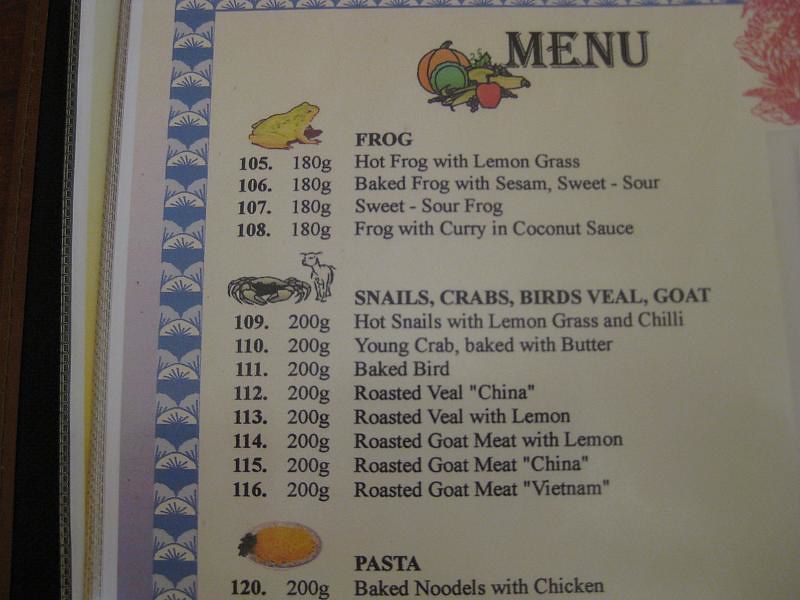This image captures a partial view of a menu with a white background, slightly off-center, featuring the name "Paul Black" in capital letters at the top. The header also includes a cartoon depiction of assorted vegetables, such as a pumpkin, apple, and squash. The section focused on frog dishes shows the word "FROG" in black letters accompanied by a yellow frog illustration. This section lists various frog dishes, including Hot Frog with Lemongrass, Baked Frog with Sea Sesame, Sweet and Sour Frog, and Frog with Curry and Coconut Sauce, each labeled with corresponding grams—105g, 106g, 107g, 108g, and 180g.

Below the frog section, the menu continues with items such as snails, crabs, birds, veal, and goat. Each type of dish includes a cartoon illustration, with examples like a crab and a goat. Similar to the frog section, these dishes also display their respective gram measurements.

Further down, the name "Paul Black" reappears above the pasta section, featuring a cartoon bowl of pasta. However, only one dish is visible in this section—Baked Noodles with Chicken, 200g, designated as number 120.

The menu seems to be coated in plastic and rests on a wooden table, as suggested by the details visible to the far left. Additionally, a red floral design decorates the upper right-hand corner of the image. The rest of the menu remains out of the frame.